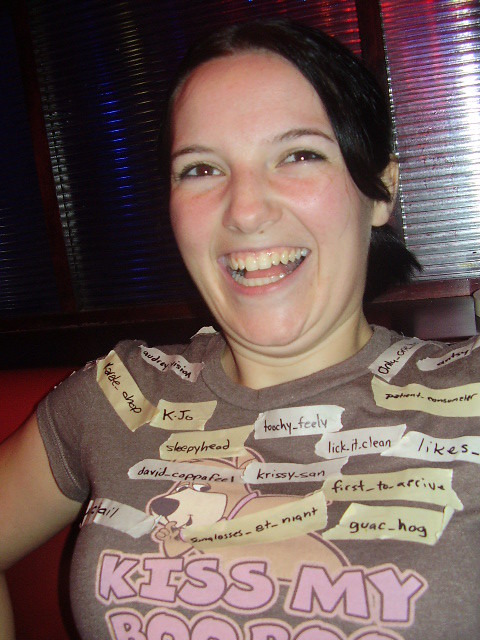In the photograph, a woman in her late 20s is captured mid-laughter, her face radiating joy. She has expressive brown eyes and black hair that's neatly pulled back. The backdrop features a window with blinds partially drawn. She is dressed casually in a gray t-shirt that features the character Boo-Boo from the classic cartoon "Yogi Bear," alongside the humorous phrase "Kiss my boo-boo." The t-shirt has a playful vibe, adding to the light-heartedness of the scene. 

Significantly, the woman is adorned with various pieces of tape covered in handwritten Instagram handles and phrases. Each piece of tape displays different quirky and playful labels such as "guac hog," "first to arrive," "Chrissy San," "lick it clean," "touchy-feely," "sleepyhead," "K-Joe," "David Coppa feel," "sunglasses at night," "something cheap," "Audrey-ism," and "only something." These humorous tags suggest an inside joke or perhaps a funny game among friends, lending an extra layer of personality and story to the image.